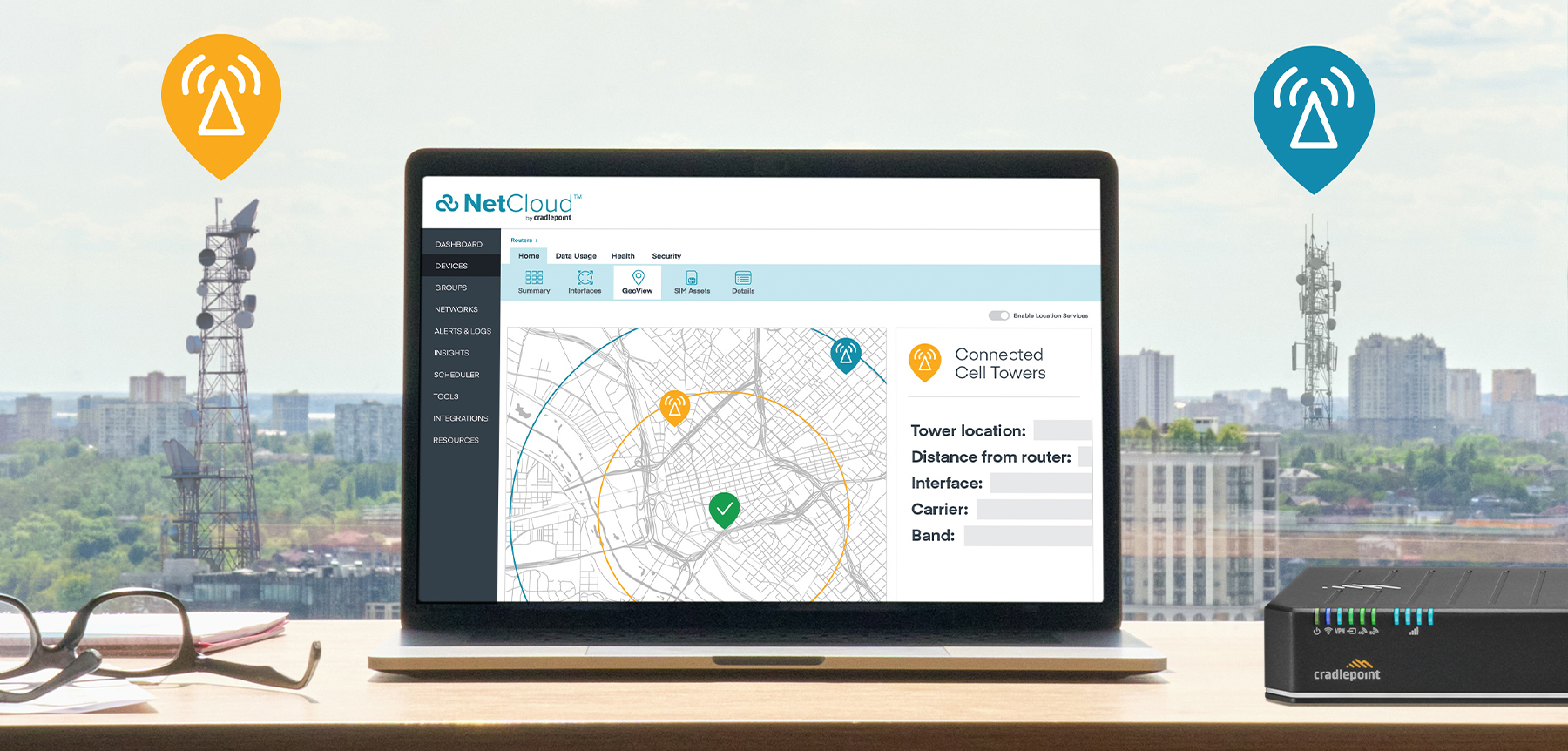The photograph showcases a laptop placed on a desk, facing a large window with a cityscape view. The city features two distinct towers visible through the window: the one on the left has an orange bubble with a white triangle and four lines suggesting noise or signal emission, while the tower on the right displays a similar symbol but in blue. Both towers seem indicative of cellular or communication infrastructure. On the desk, there are glasses lying upside down, a sheet of paper, and a router in the bottom right corner. The laptop screen displays a webpage from NetCloud, featuring a map highlighting connectivity details, such as 'Connected Cell Towers', 'Tower Location', 'Distance from Router', 'Interface', 'Carrier', and 'Band'. A green checkmark within a circle marks the location on the map. The detailed setup and symbols suggest the photo is an advertisement for NetCloud, emphasizing their service's ability to provide connectivity and detailed information about nearby cell towers.